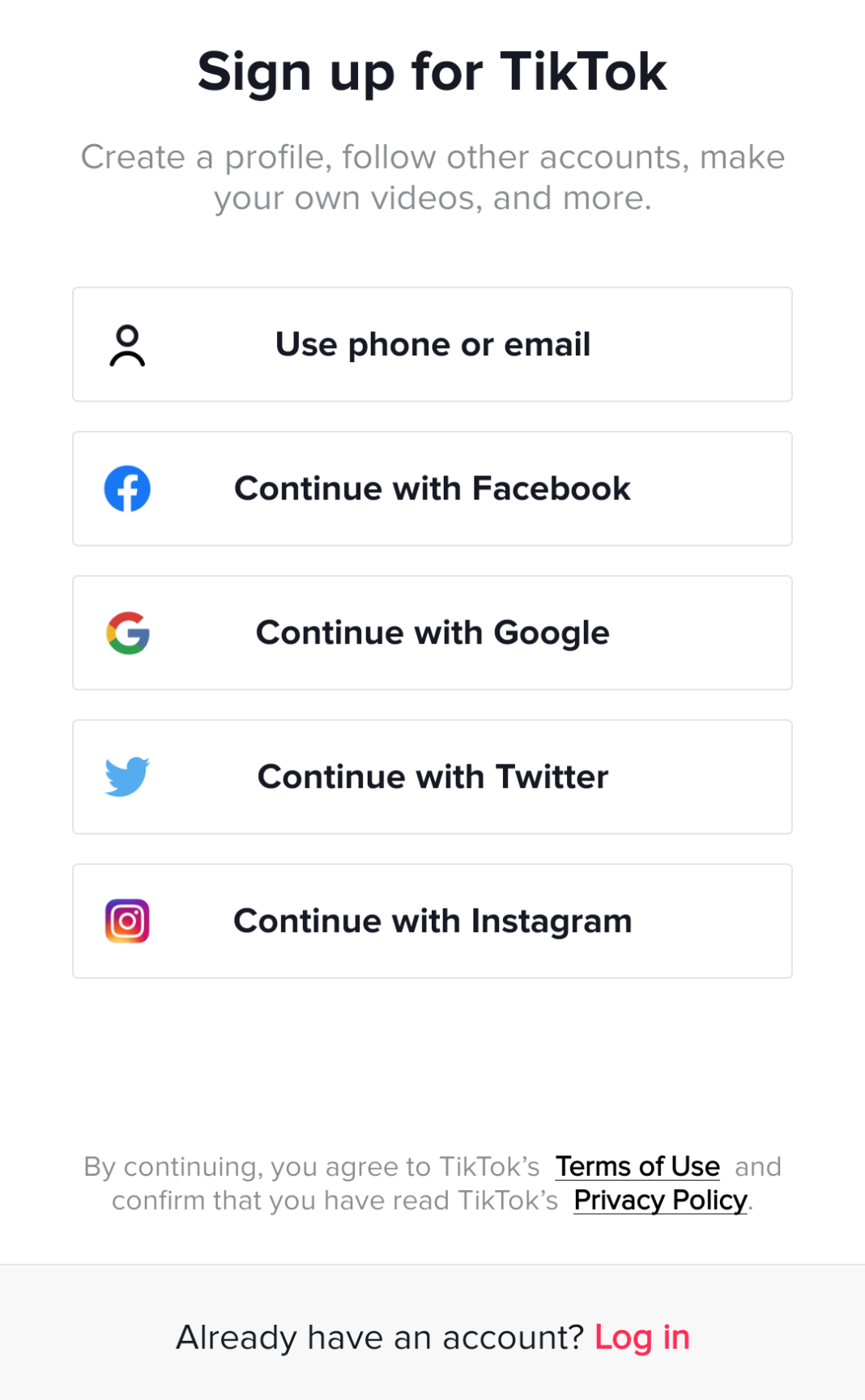This image provides a comprehensive overview of the sign-in and sign-up options available for TikTok. It guides users through the process of creating a profile, following other accounts, and making their own videos, among other features. Users can choose to sign up or log in using various methods: via phone or email, or by continuing with third-party platforms such as Facebook, Google, Twitter, or Instagram. Each of these options is represented by their respective logos for easy identification. The image also mentions that by continuing the sign-up process, users are agreeing to TikTok's terms of service and confirming their understanding of the platform's privacy policy. For those who already have an account, there's a prompt to log in, highlighted in red text.